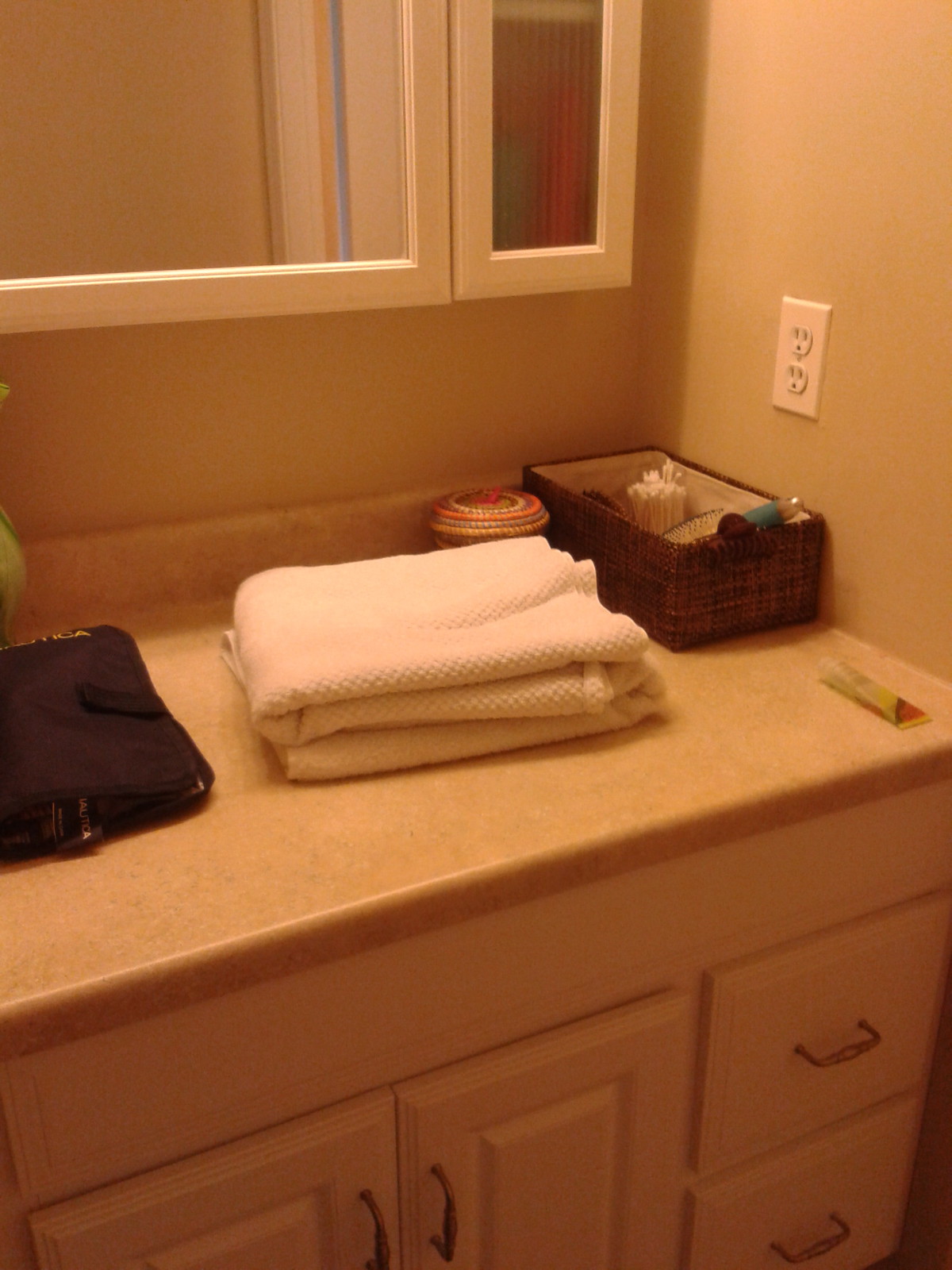The image depicts a neatly organized bathroom with a predominantly beige color scheme. The beige walls blend seamlessly with the beige countertop, which features light-colored drawers adorned with handles that are slightly darker than the cabinets themselves. A double wall socket is positioned conveniently on the wall, ideal for plugging in appliances such as a blow dryer.

On the countertop, a few neatly folded white towels are positioned towards the center. To the right of the towels sits a wicker basket filled with various items, including identifiable Q-tips among other indistinguishable objects. Adjacent to the basket is a small jar with an orange lid, placed between the towels and the wicker basket.

To the left of the towels, there's a black fold-up holder fastened with velcro, though its contents are not visible. Behind the towels, a mirror is mounted above the countertop, hinting at a dual-section storage area with a small and a main section. The overall ambiance of the image is neutral and monochromatic, dominated by shades of beige.